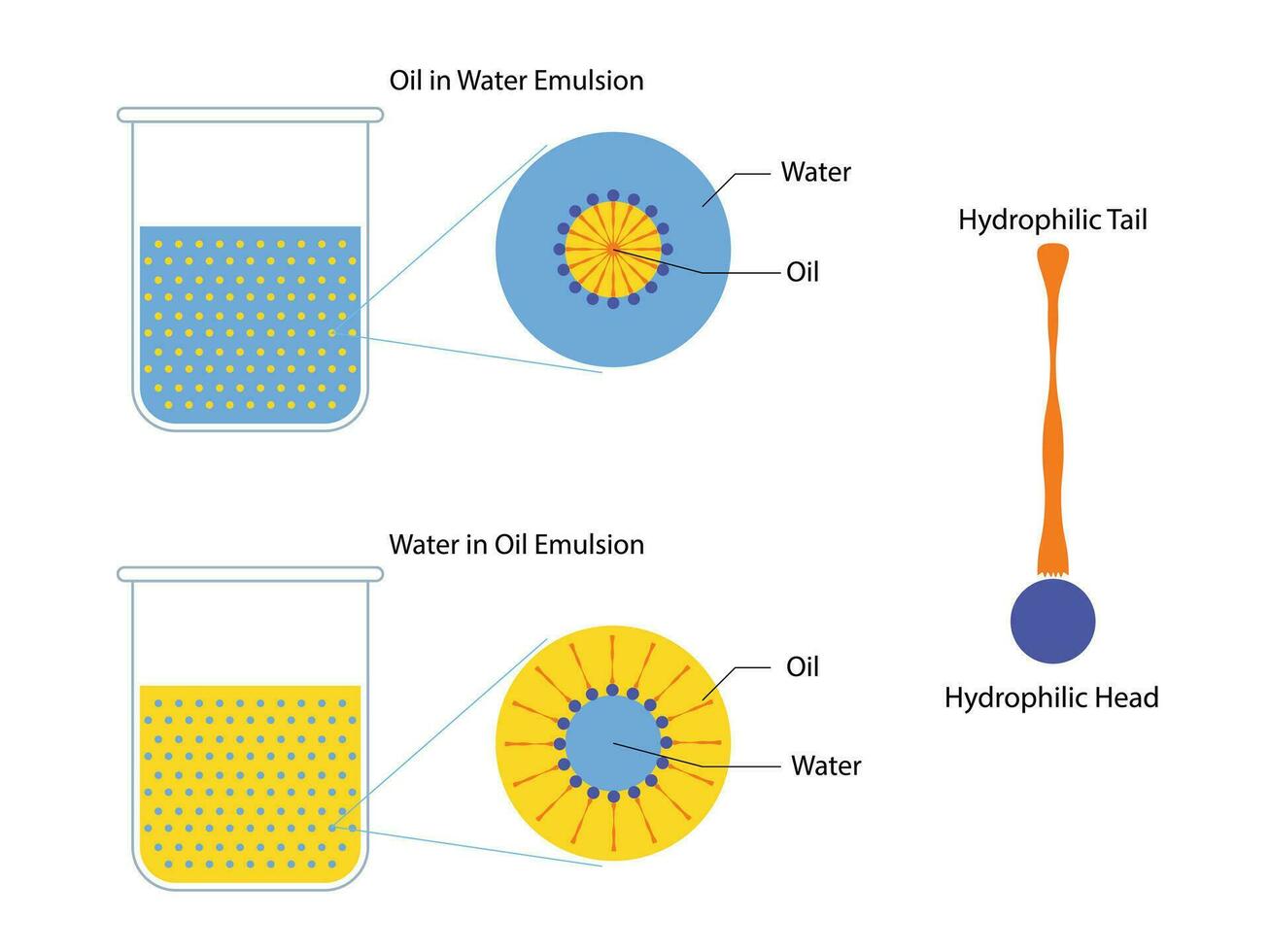This scientific diagram features illustrations of oil-in-water and water-in-oil emulsions. At the top left, a beaker filled with a blue liquid containing yellow dots is labeled "oil in water emulsion." Emanating from one of the yellow dots, two lines reveal a magnified view of the dot, showing an inner yellow circle labeled "oil" with spikes ending in dark blue dots (hydrophilic heads) and red lines extending from the center (hydrophilic tails), all encased in a larger blue circle labeled "water." Below, a similar beaker filled with a yellow liquid and blue dots is labeled "water in oil emulsion." Here, the blow-up view shows a large yellow circle labeled "oil" surrounding a smaller blue circle labeled "water," with red lines extending from the blue circle's center through dark blue dots at the outer edge. On the right side of the diagram, a close-up illustration labels a red line as the "hydrophilic tail" and a blue dot as the "hydrophilic head."